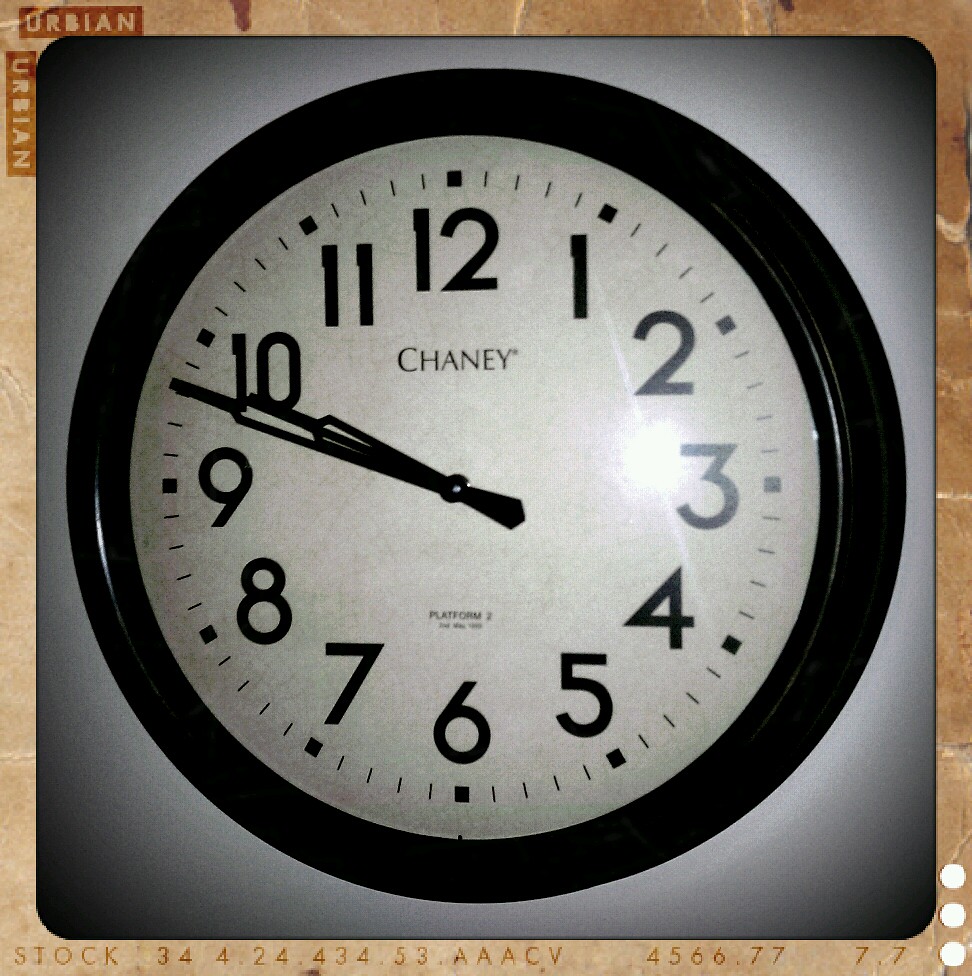This photograph captures an analog wall clock with a classic, vintage aesthetic. The round clock features a black frame encircling a white clock face, adorned with black numbers. Each hour is marked by a black square, with smaller lines in between to indicate the minutes. Below the 12 o'clock position, the name "Chaney" is prominently displayed in black text, suggesting the brand of the clock. The clock shows a time of approximately 9:48, indicated by its black hour and minute hands, though it lacks a second hand. The wall behind the clock is gray, and the clock is mounted on a border with a brownish tone that features the text "URBIN" in the upper left-hand corner. At the bottom of this border, it reads "stock 344-244-3453," with three holes punched into the bottom right-hand corner, adding to the vintage filmstrip-like appearance. The scene is illuminated by artificial light, perhaps suggesting a nighttime setting. The overall look and design hints that the clock might be from the 1940s, enhancing the nostalgic feel of the image.